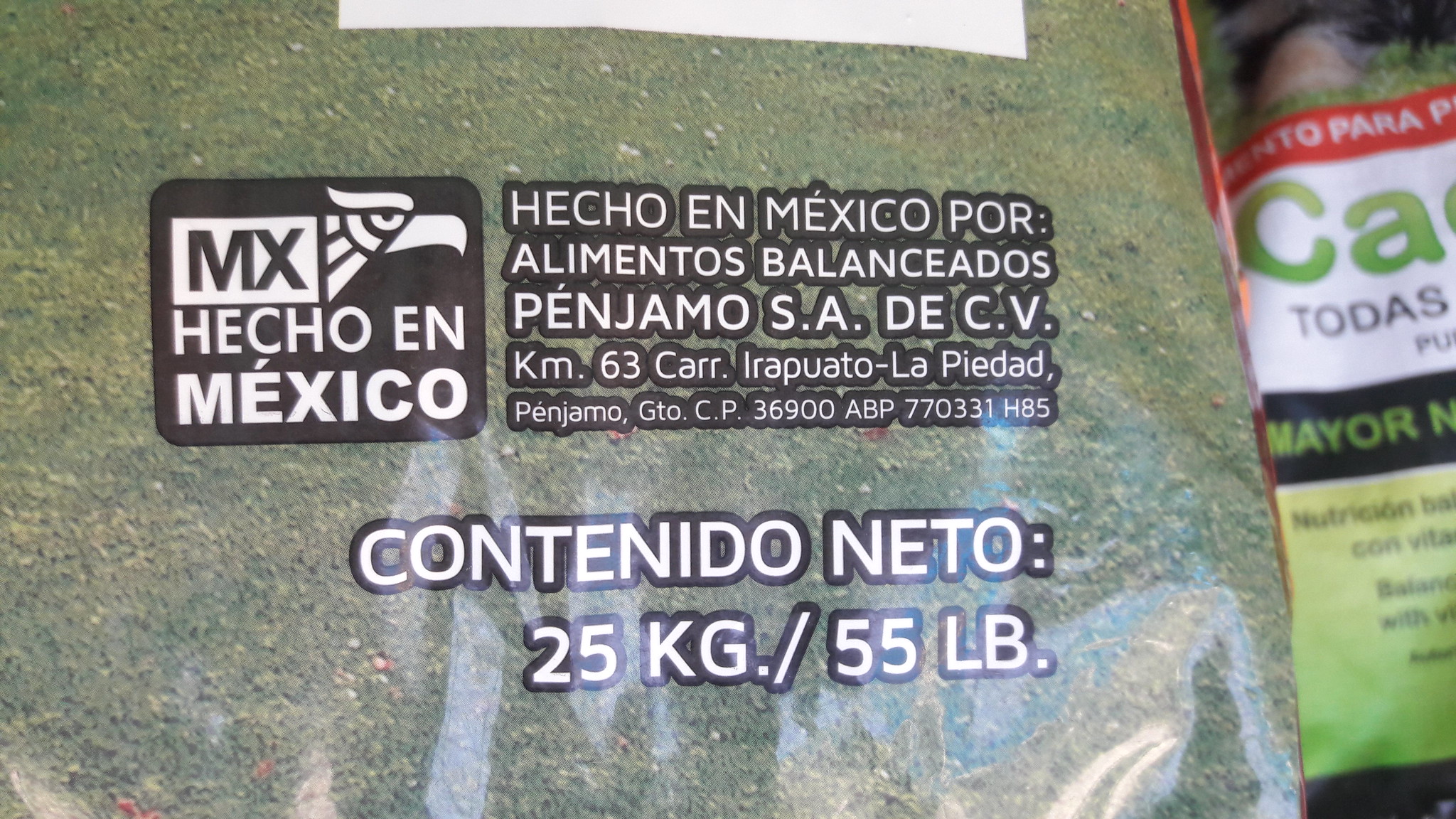This image features a packaged food item, presumably made in Mexico, as indicated by the text "Mexico Jekyll and Mexico" on the container. The packaging is black with white writing and includes nutritional information, suggesting it is an edible product. The backdrop for the container is a neutral greenish color. To the right, there is a bright green packet adorned with a red stripe and large green capital letters, likely displaying additional product details or branding. The overall composition juxtaposes the subdued tone of the background with the vibrant colors of the packaging, drawing attention to the food items.